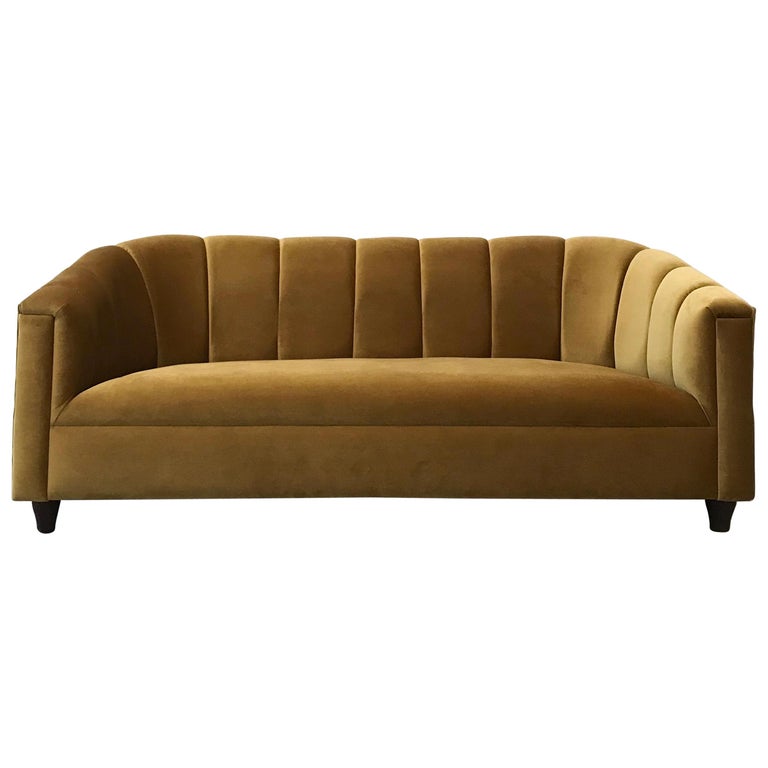This image showcases a vintage-style sofa presented against a completely white background, reminiscent of a product photo on a furniture retailer's website. The sofa, with a golden tan fabric, features dark wooden, wedge-shaped legs that give it a suspended appearance as if it’s floating. The front view reveals a rectangular, poofy seat cushion and a lower backrest that's divided into several vertically seamed sections for a decorative effect. The high arms and rounded top edges add to its classic yet contemporary design.